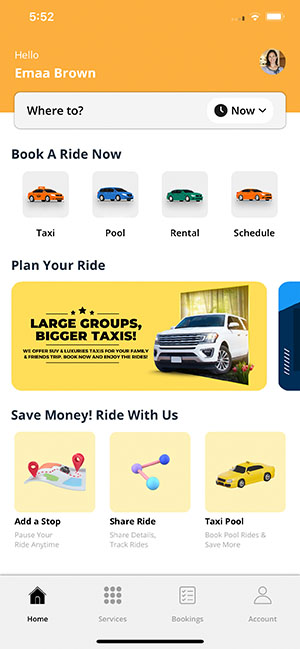The image prominently features an app interface for booking rides, titled "Hello, EMAA Brown." The interface includes a header with the name "EMAA" spelled out clearly. Below the header, there is a prompt asking "Where to?" and an option to "Book a Ride Now,” with various options such as taxi, pool, rental, or schedule.

Further down, it encourages users to "Plan Your Ride," illustrated through a series of icons and text graphics. These graphics highlight the benefits of using the service, like saving money, adding a stop, sharing rides, and different ride options such as taxi or pool.

The image itself prominently displays a large white vehicle, which is situated next to what appears to be a PC tower. To the right of the car, the text promotes services for large groups, emphasizing the availability of bigger taxis and luxurious options suitable for family and friends’ trips. There is also a call to action encouraging viewers to "Book Now." Some parts of the text are unclear, but the overall message revolves around the convenience and variety of ride-booking options available through this service.